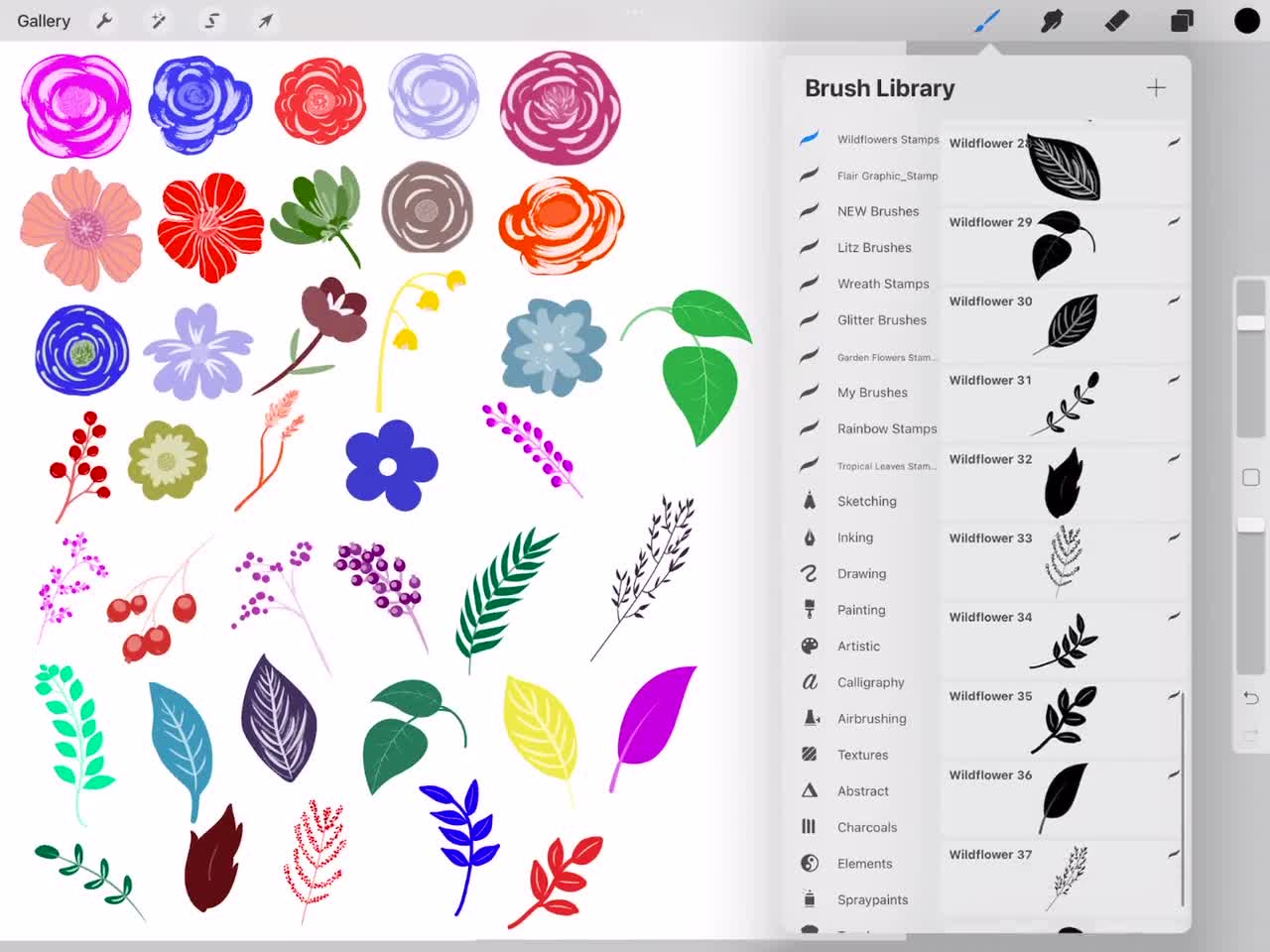The image is a rectangular screenshot, approximately five to six inches wide and four inches high, of a computer program on a tablet, likely an iPad. The left side is open with no border, while the top and bottom have thin gray borders; the top border includes the word "Gallery" and several icons, including a wrench, a pen, a zigzag line, and an arrow. The right side has a blue paintbrush icon, followed by a black paintbrush, possibly an eraser, some paper icons, and a black circle. 

The main area of the screen has a white background displaying seven rows of multicolored flower patterns in a grid format. The first four rows display various types of flowers in different colors, while the bottom rows showcase leaves and berries. 

On the right side, a drop-down menu is visible with the label "Brush Library" at the top. This menu is divided into two columns. The left column lists different categories of brushes such as sketching, inking, drawing, painting, artistic styles, and features "wildflower star tips" at the top. The right column illustrates black-and-white images of wildflowers, numbered 28 to 37, mimicking stamp designs. The wildflowers on the right column match the colored versions displayed on the main white area of the screen. The detailed layout and the juxtaposition of colored and black-and-white flower designs underline the creative tools and options available within the program.